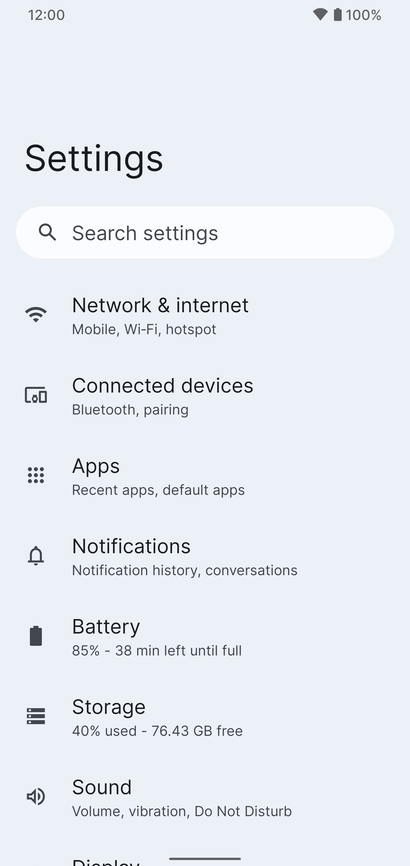The image is a detailed screenshot from a smartphone, featuring a very light blue background, including the top header. On the top left, the time is displayed as 12:00. On the top right, there is a battery icon indicating a full charge at 100%, and to its left, the Wi-Fi icon is visible, resembling an inverted triangle.

Centered towards the left side of the image, the word "Settings" is prominently displayed in large, black font. Below this, there is a search box represented by a long, white rectangle with rounded corners. Within the search box, on the left end, there is a circular magnifying glass icon, and the text "Search settings" is written inside the box.

Below the search box, a list of menu items is presented, each accompanied by an icon. The list includes:

1. "Network & Internet" with sub-options for 'Mobile, Wi-Fi, Hotspot'.
2. "Connected devices".
3. "Apps & notifications".
4. "Battery".
5. "Storage".
6. "Sound".

The top of the next item is barely visible, likely indicating the word "Display".

This structured and concise layout within the settings menu facilitates easy navigation and quick access to various phone settings.